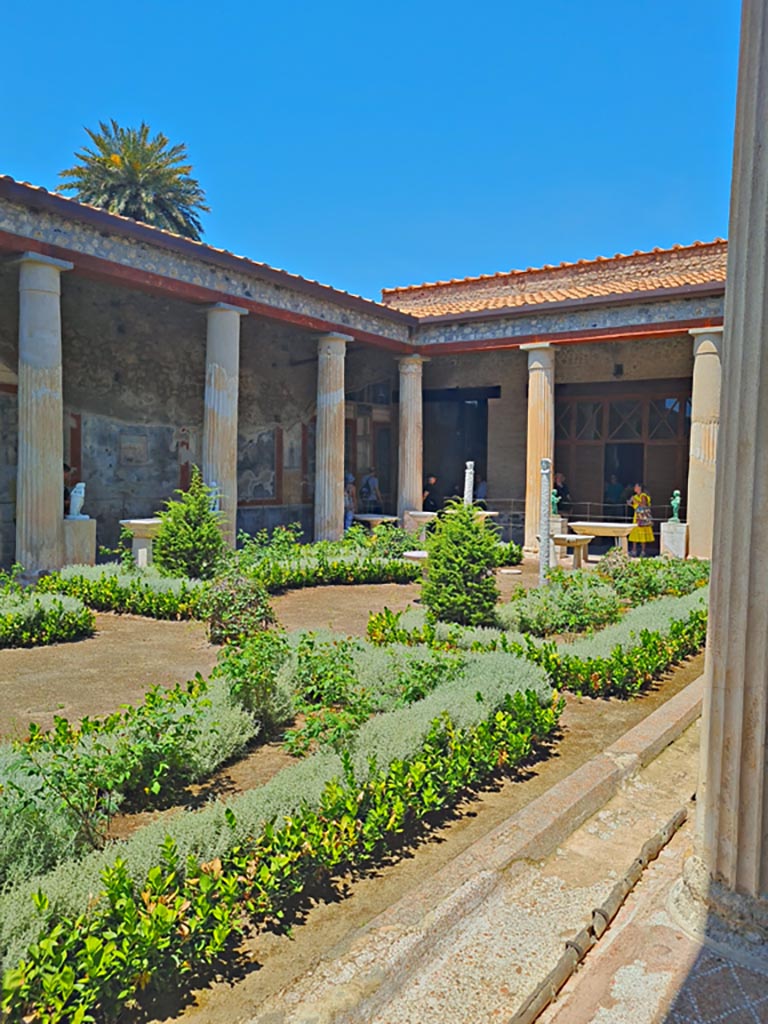The image depicts a large, seemingly abandoned building with an architectural design reminiscent of a Spanish villa. The structure features an open courtyard at its center, surrounded by walkways and columns. The walls of the courtyard are heavily weathered, adorned with faded pastel painting in colors such as light green, maroon-brown, beige-yellow, and bluish-gray, which are chipping away to reveal gray concrete or repair work underneath. 

On the left side of the courtyard, a wall with yellow and red painted squares stretches along a walkway, with patches of the paint missing. The walkway, composed of pavers or stone, runs under a roof supported by Romanesque columns with distinct grooves. These columns form a square on the right side of the image. A small metal wire fence, held up by posts, encircles the garden in the courtyard center, where healthy green plants grow. 

Above the courtyard, you can see the sky with a palm tree silhouetted in the background. The building has an orange or terracotta tiled roof, adding to its Spanish architectural style. Despite the apparent neglect, the courtyard garden remains vibrant, indicating that the space may still receive some care. The overall feel suggests that this building might once have served a grander purpose, possibly as a school or museum, given its size and decorative details.